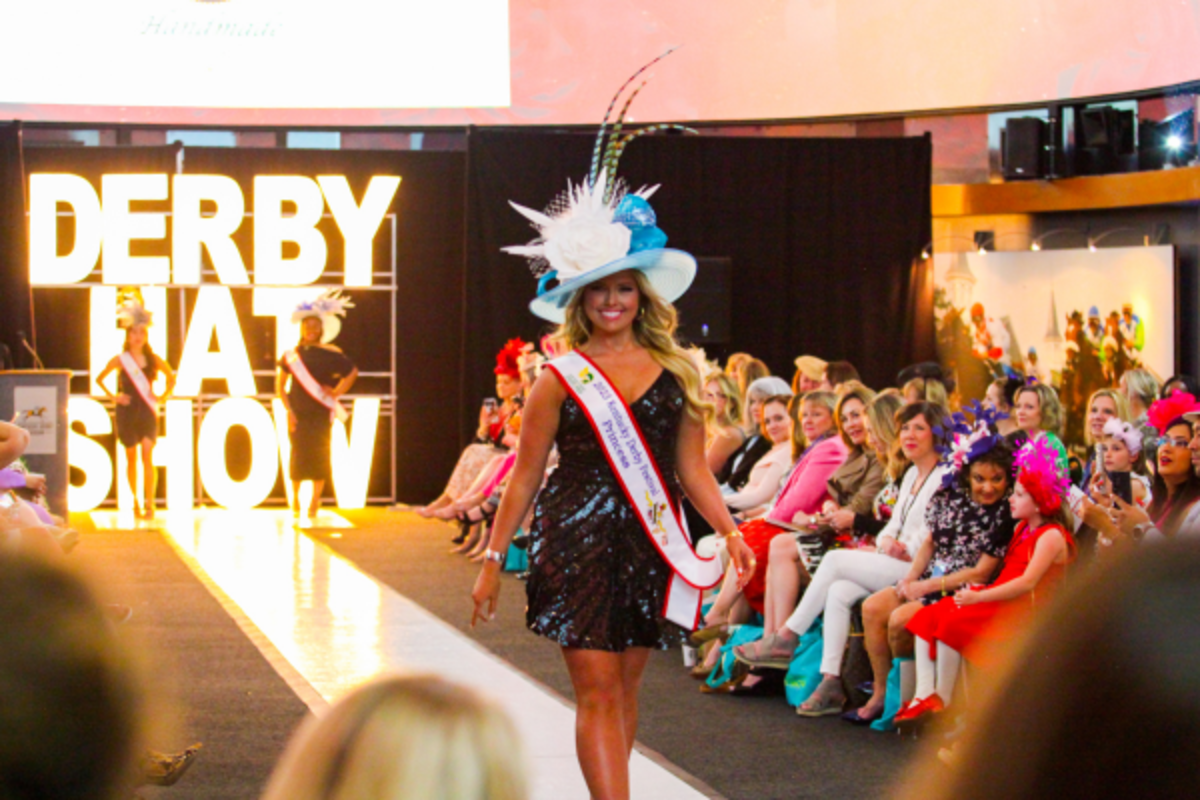The captivating photo captures a moment from the Derby Hat Show, evident from the large illuminated letters in the background that spell out "Derby Hat Show." Center stage, a striking blonde model with a warm tan parades down the runway, embodying elegance and flair. Her voluminous long, curly hair complements a grand, light blue hat adorned with an oversized white flower and delicate feathers jutting from the top. Clad in a sleeveless, glittery black mini-dress, she exudes confidence and charm. A white sash with a red border drapes diagonally across her front, inscribed with blue text that reads "2023 Kentucky Derby Princess." Smiling radiantly at the audience, she captures the crowd's admiration. The audience primarily consists of women dressed in vibrant attire, enthusiastically watching the event from their seats. In the background, two other models wait for their turns, flaunting their own intricate hats, adding to the pageantry of the Derby Hat Show.